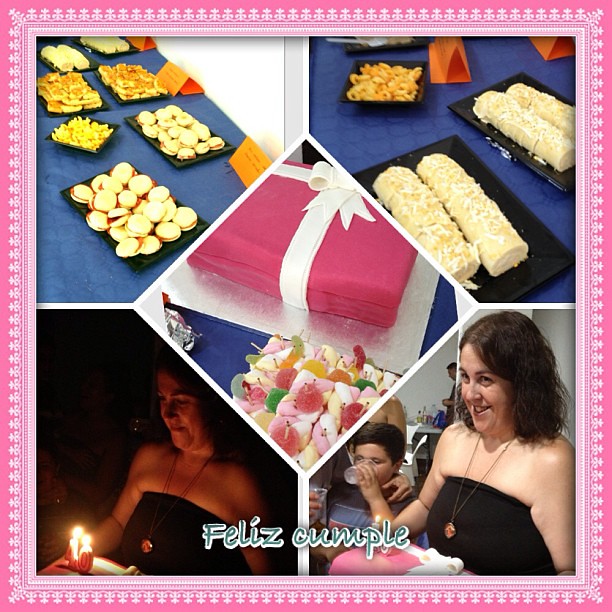The image is a collage of five photos, bordered by a pink frame adorned with white star-like details. The collage features two photos at the top, two at the bottom, and a diamond-shaped photo in the center. The top left photo displays an assortment of finger foods on a table with a blue tablecloth and orange place cards identifying the dishes. The upper right photo also showcases more food items, including cream-colored rolls on black rectangular plates. In the center diamond-shaped photo, there’s a close-up of a cake wrapped like a present, pink with a white bow, surrounded by candies. The bottom left photo captures a woman in a dark silhouette, dressed in a black tube top, holding a birthday cake with lit "40" candles. The lower right photo shows the same woman smiling brightly, with a little boy drinking from a glass next to her. The collage as a whole appears to celebrate a birthday, with the phrase "Feliz Cumple" visible at the bottom center.